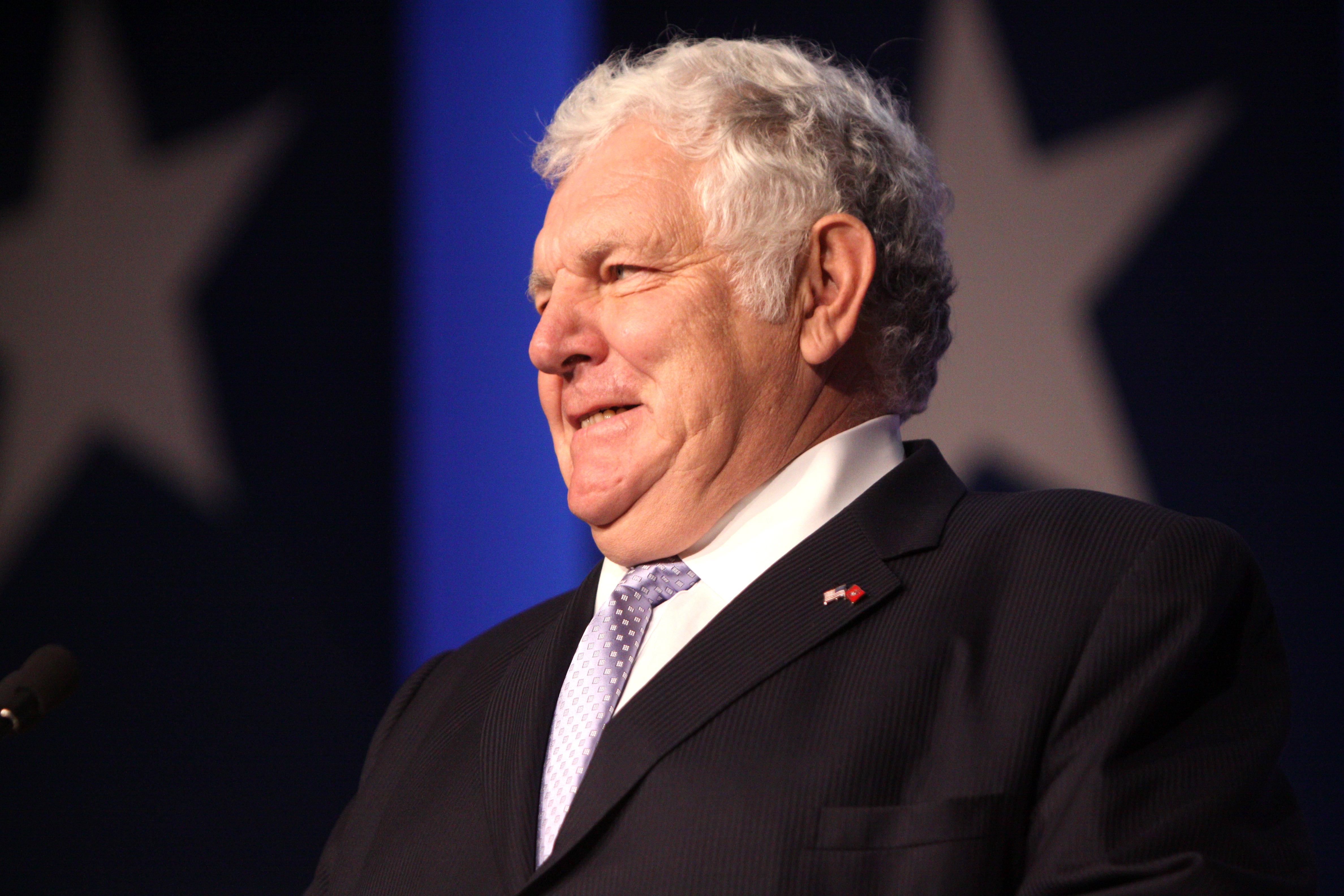In the image, an elderly man appears in a color close-up photograph. He is largely overweight, with a chubby face, a big double chin, and a large ear. His short, wavy hair is a mix of gray and white, suggesting he could be around 65 to 70 years old. He is wearing a dark black suit paired with a white-collared shirt, and a blue tie adorned with white polka dots. The suit jacket also features an American flag pin and another small, red pin that is difficult to identify. The man has a tense, unsmiling expression, adding to the serious tone of the photograph.

In the background, two vertical blue stripes with white stars are visible, along with what appears to be American flags or similar signage, adding a patriotic atmosphere. On the left-hand side of the image, the black top of a microphone can be seen, hinting that the man might be standing on a stage, possibly at a political event or convention, either preparing to speak or listening to someone. The dark backdrop contrasts with the man's figure, making him the focal point of the photograph.